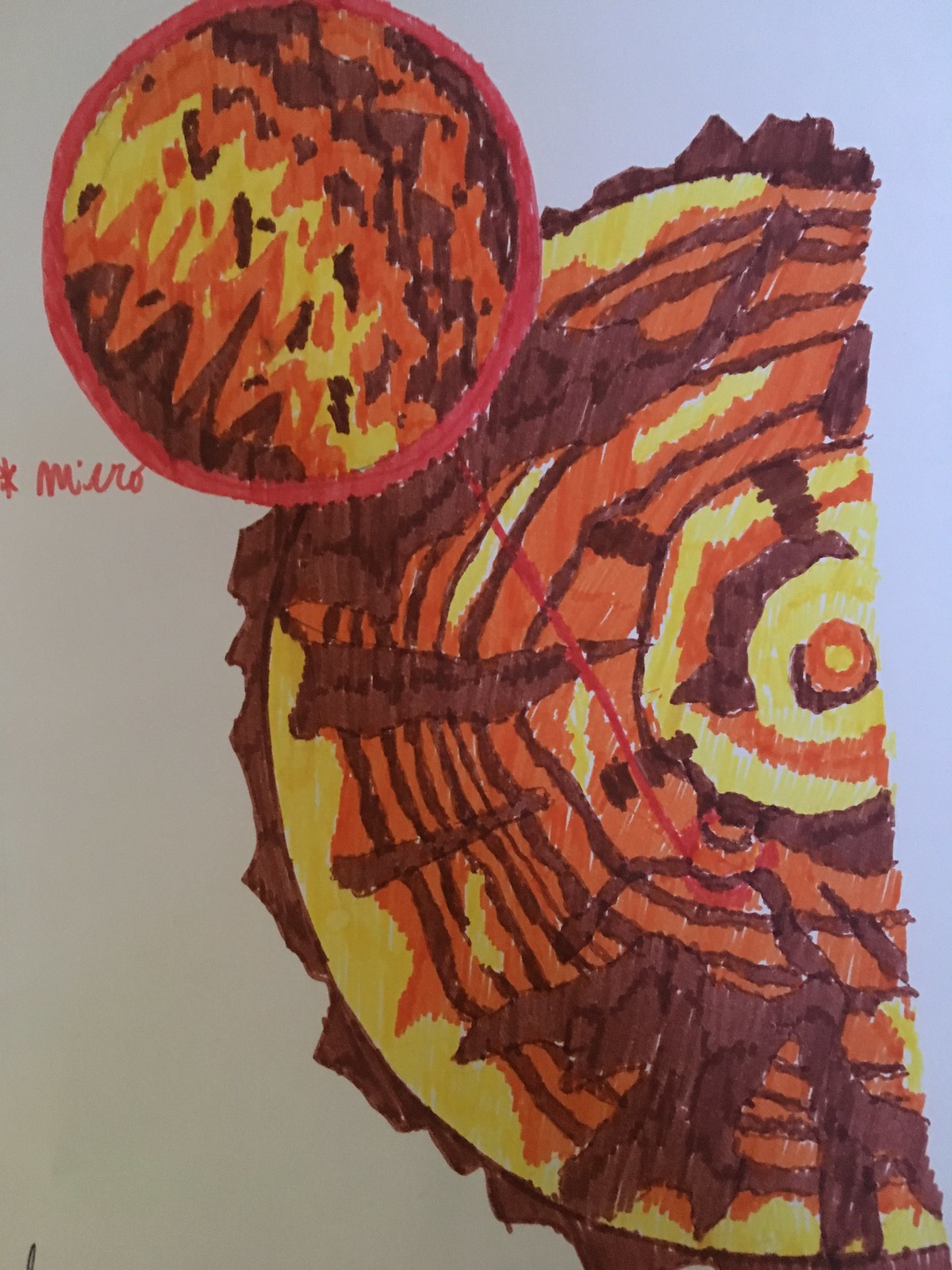This is a child's detailed art project depicting a tree stump, viewed from above, showcasing its intricate growth rings. The stump's concentric rings are meticulously illustrated using a thick brown marker, with selected rings highlighted in vibrant orange and the entire stump colored with yellow, creating a rich tapestry of orange, yellow, and brown hues. Radiating cracks extend from the outer edges towards the center, drawn in brown with black inserts, adding depth and realism to the piece. Encircling the stump is a dark brown bark. Notably, there's an emphasis circle outlined in red, containing the word "Miero" written beneath it in cursive, possibly representing a close-up of one of the rings. This smaller red circle, filled with squiggly yellow and brown lines, sits prominently within the larger context of the stump. The background is split, with a gray hue on the left transitioning to a light blue on the right, framing the artwork. Altogether, this project balances abstract and realistic elements through its detailed portrayal of the tree rings and the colorful application of markers.